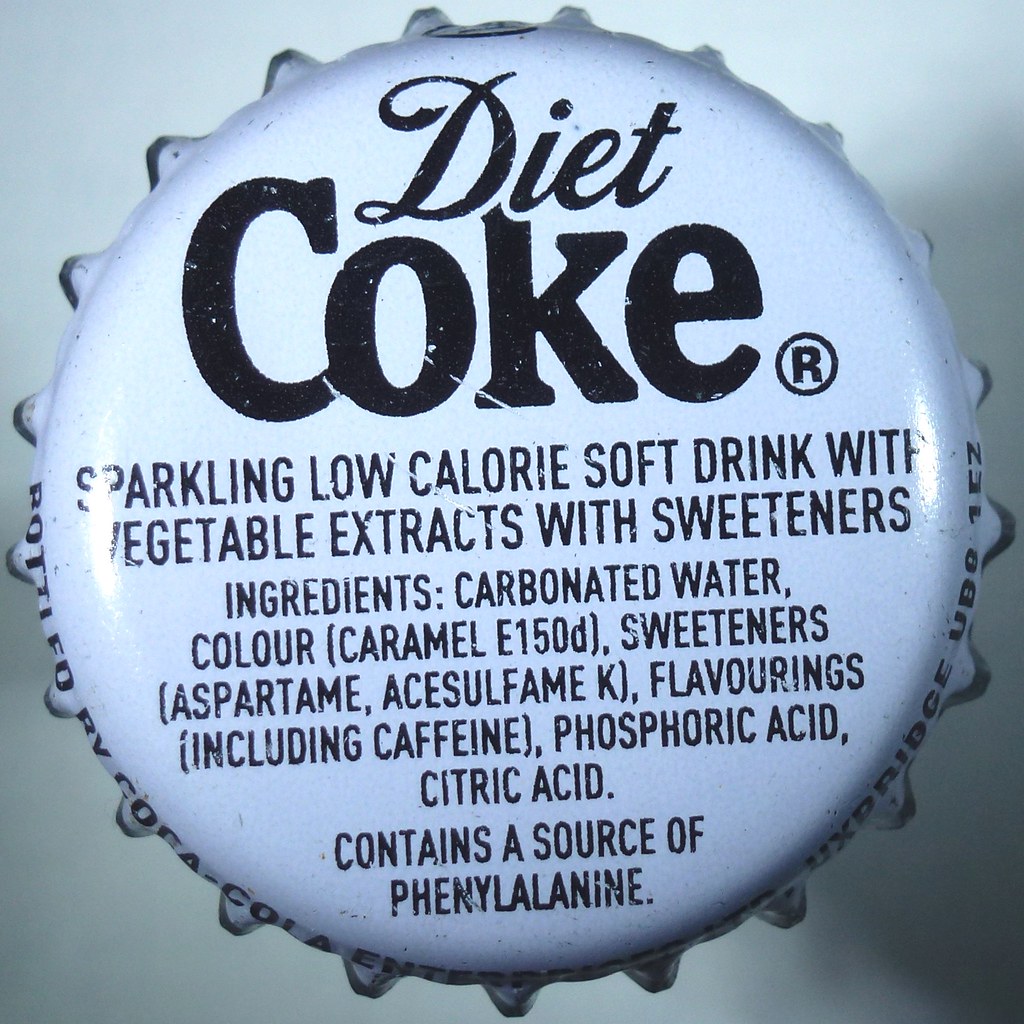This detailed close-up image showcases the top of a Diet Coke bottle cap. The cap is silver and rests on a white background, casting a subtle shadow. Prominently displayed at the top in black print is the classic "Diet Coke" logo, accompanied by the registered trademark symbol. Below this logo, the text reads: "Sparkling Low-Calorie Soft Drink with Vegetable Extracts with Sweeteners." Further down, the cap meticulously lists the ingredients: "Carbonated Water, Color (Caramel E150D), Sweeteners (Aspartame, Acesulfame K), Flavorings (including Caffeine), Phosphoric Acid, Citric Acid," and it notes that it "Contains a Source of Phenylalanine." Around the sides of the cap, which are partially obscured in the shadow, there are additional details indicating that the product is bottled by Coca-Cola, followed by some numbers and letters. The cap features a textured edge, typical of bottle caps, with small bumps encircling its circumference.